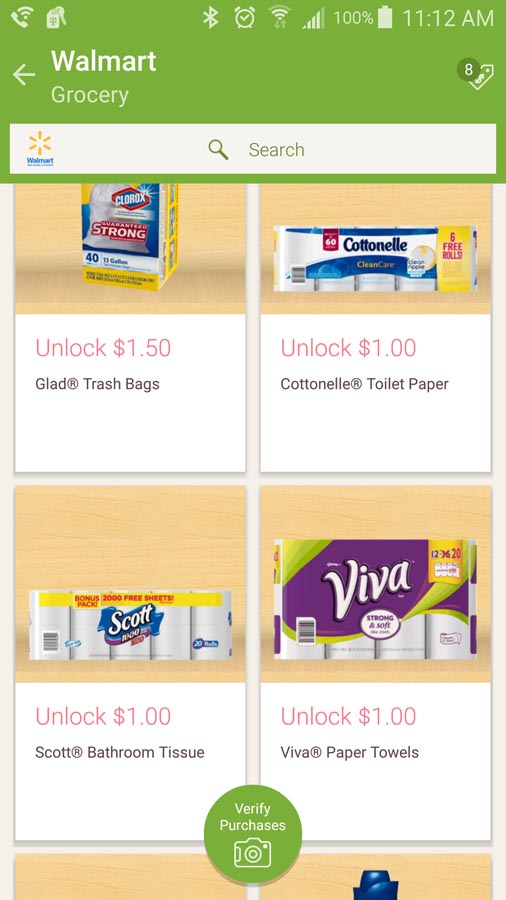At 11:12 AM, a screenshot from the Walmart grocery app displays a fully charged battery and an alarm clock symbol. The image features a search bar and a price tag reading $8.00. Four grocery items are listed with "Unlock" promotions displayed in red text: Clorox trash bags for $1.50, Cottonelle toilet paper for $1.00, Scott bathroom tissue for $1.00, and Viva paper towels for $1.00. Additionally, a green circle with a white camera icon is visible, indicating verified purchases.